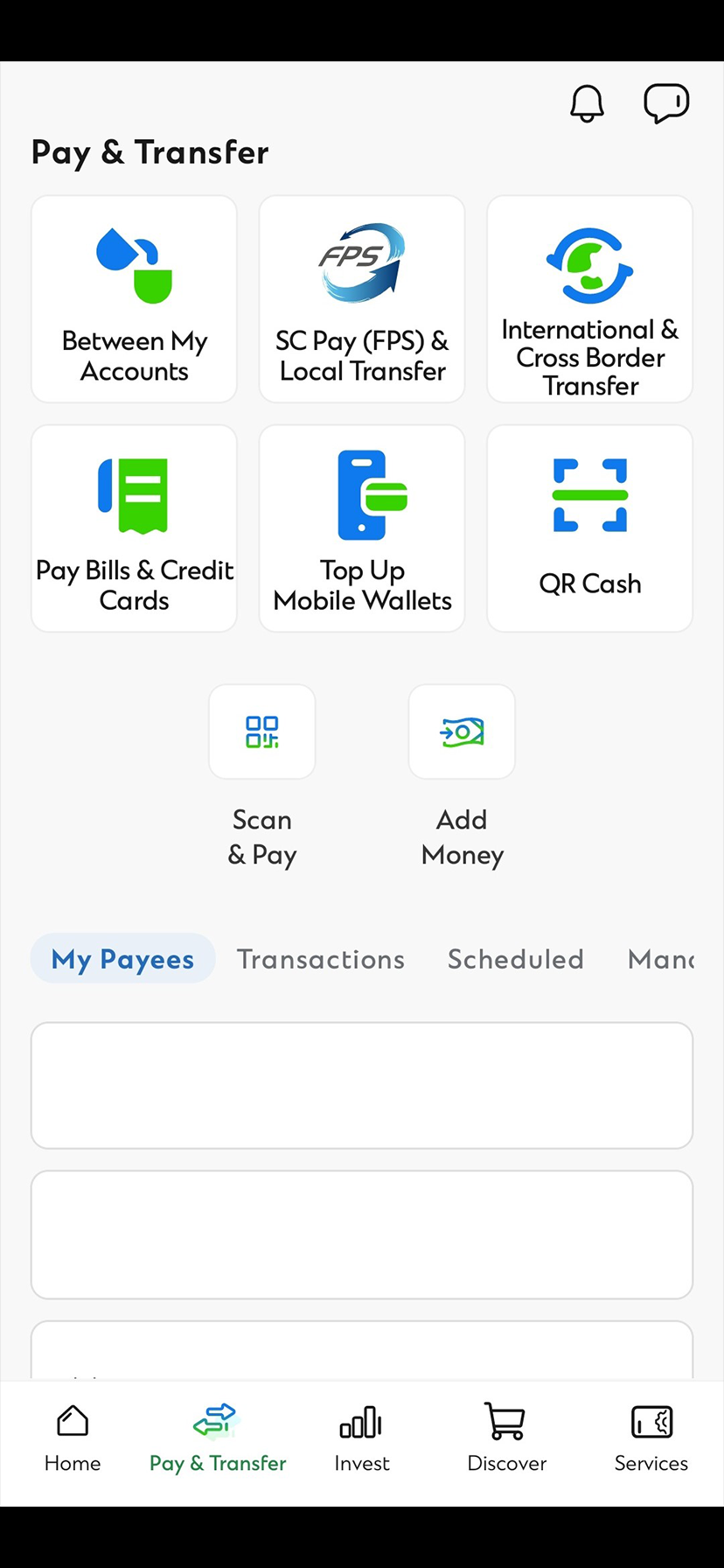A detailed image description of a mobile money transfer app interface:

The image showcases a mobile money transfer application displayed on a vertically oriented device. The screen has notable black bars, approximately one inch thick, at the top and bottom edges. The app interface sits on a gray background. At the very top in black font, the text reads "Pay and Transfer." To the right, there are two icons: a message icon likely for live chat support and a notification icon.

Beneath this header, the main area of the screen is divided into six white, rectangular sections, each containing distinct transfer and payment options. The sections are labeled as follows:

1. "Between My Accounts," illustrated with two cups pouring water into each other.
2. "SCPay, FPS and Local Transfer."
3. "International and Cross-Border Transfer."
4. "Pay Bills and Credit Cards."
5. "Top-Up Mobile Wallets or QR Cash."
6. "Scan and Pay" or "Add Money Here."

Further down, the interface provides additional navigation options listed as "My Payees," "Transactions," and "Scheduled."

At the very bottom of the screen, there are five selectable menu options: "Home," "Pay and Transfer," "Invest," "Discover," and "Services."